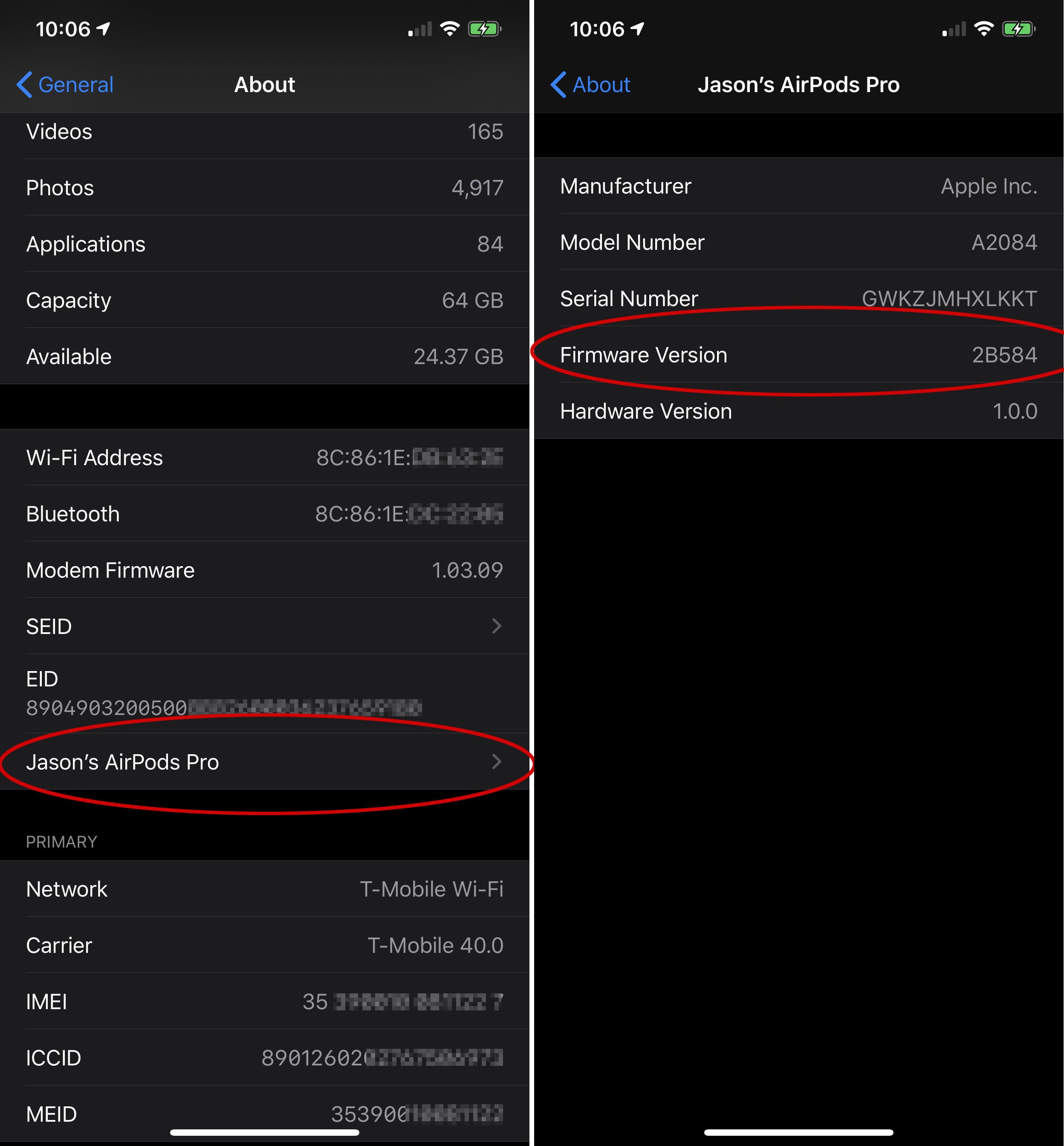Here's a cleaned-up and detailed caption:

---

**Detailed Device Information Screen**

The image features a screenshot of a smartphone’s "Settings" menu with a focus on "General" settings. On the left side of the screenshot, the "About" section is displayed, showing critical details such as the storage capacity, available space, and Wi-Fi address. Notably circled in red is "Jason's AirPod Pro," highlighting a connected device.

On the right side, the continuation of the "About" section reveals additional technical specifications, including the network provider, carrier information, manufacturing model, serial number, firmware version, and hardware version. The entire screen has a black background, providing a stark contrast to the white text and the red circle emphasizing important information.